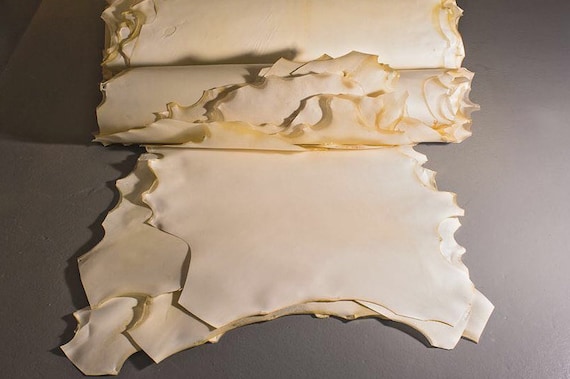The image is a color photograph oriented in landscape format. It depicts a close-up of several creamy beige cloth-like sheets, possibly handmade paper, parchment, or pasta sheets, arranged on a gradient gray background, which transitions from darker on the left to lighter on the right. In the foreground, there are roughly six sheets of this material, stacked haphazardly upon each other. Their irregular, jagged edges are a golden brown color, suggesting a handmade or torn appearance. In the middle of the image, one section of the material is rolled up, resembling a rolling pin, with slightly pointed ends. This rolled portion and the stacked sheets are the primary focus of the image. The lighting is natural and illuminates the image clearly, enhancing the detailed textures and color variations of the material. The overall composition suggests a sense of realism, with no other objects or people present in the frame.